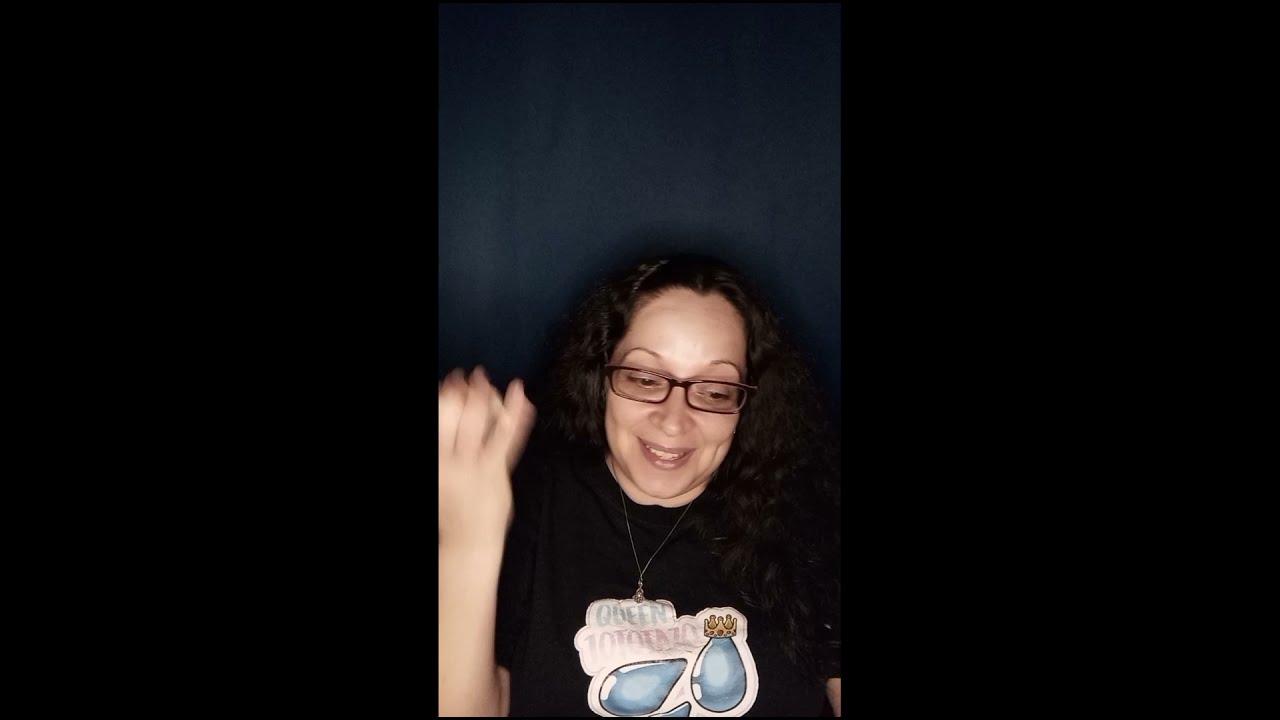The photograph features a woman standing against a dark gray background on the left side of the image, with an all-black panel on the right side. She is in her late 40s to early 50s, has long, dark brownish-black wavy hair, and is looking down. The woman is wearing maroon-framed glasses and thin, arched eyebrows. Dressed in a black t-shirt, she has a necklace with a silver teardrop pendant. The t-shirt includes the text "Queen Loto Tazo" with two blue teardrop shapes beneath it, one of which is depicted with a crown. The image appears to have been taken mid-motion, as her hand is blurred and raised, possibly in a wave or gesture. She also seems to be smiling.